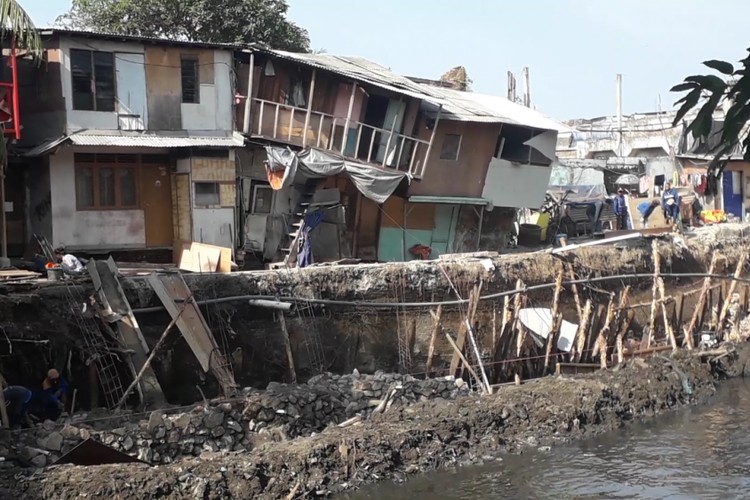The image depicts a long, outdated building resembling attached houses or apartments, situated near water. The structure appears significantly damaged, likely from a storm or river flood. The left portion of the building remains mostly intact, while the right section has collapsed and leans precariously, revealing shattered foundations. The foreground features a muddy area with loose wooden sticks scattered about, possibly debris from the damaged building. There's a barrier holding back the land from the water, which is brown and rippling. The scene is illuminated by sunlight under a very light blue daytime sky, adding a stark contrast to the overall devastation. Flags are visible on the building's side, contributing to its worn and decrepit appearance, as if the scene belongs to a less developed region.